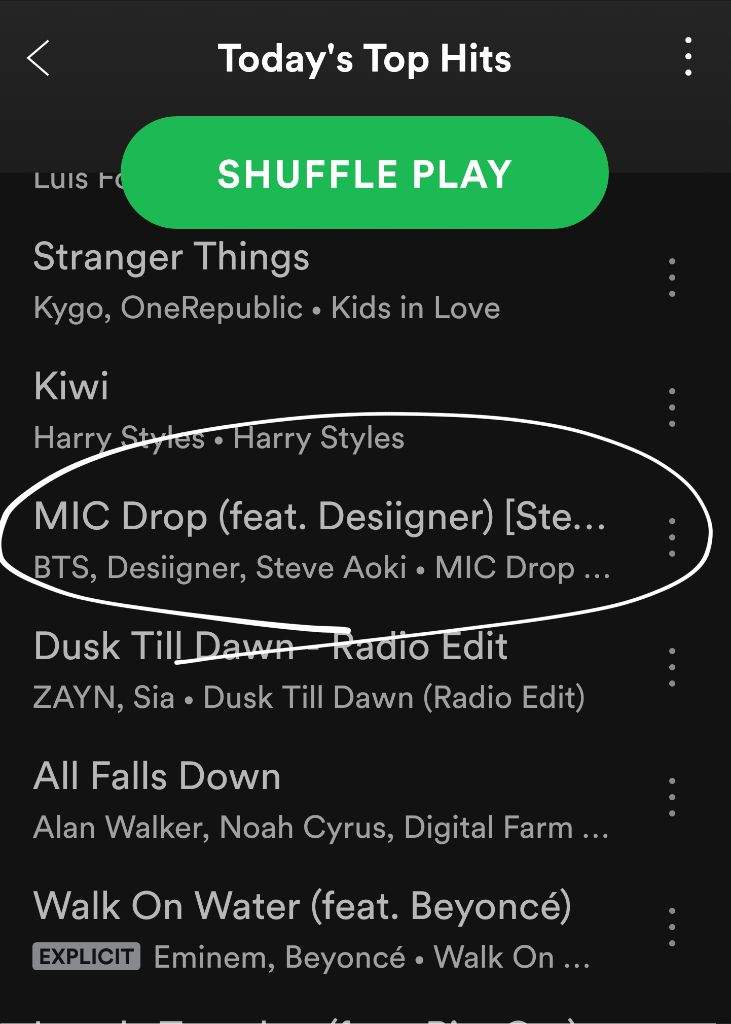**Caption:**

This image is a screenshot from a music app in portrait mode, likely viewed on a mobile device. The background is solid black with all text displayed in white. At the center top of the screen, the title "Today's Top Hits" is prominently featured. To the right of this title is a three-dot stacked menu icon, suggesting additional options, while on the left, there is a left-pointing back arrow for navigation.

Below the title is a large, elongated oval green button with the text "SHUFFLE PLAY" in all caps, indicating that the user can shuffle play the songs on this playlist. Partially obscured by this button is what appears to be the user's name, "Luis," though the full name is hidden.

The playlist consists of six songs, each with a three-dot icon to the right, possibly for additional menu options. One song stands out, as it is circled in white: "MIC Drop (feat. Desiigner) [STE...] - BTS, Desiigner, Steve Aoki." The truncated "STE..." likely references Steve Aoki.

The remaining songs on the playlist include:

1. "Stranger Things (with OneRepublic) [Kids in Love]" by Kygo.
2. "Kiwi [Harry Styles]" by Harry Styles.
3. "Dusk Till Dawn [Radio Edit]" by Zayn, Sia.
4. "All Falls Down" by Alan Walker, Noah Cyrus, Digital Farm Animals.
5. "Walk on Water (feat. Beyoncé) [Explicit]" by Eminem, Beyoncé.

Each song title includes the artist's name and, in some cases, album names or additional descriptors in brackets or parentheses. The last song, "Walk on Water," is marked as explicit with an "Explicit" label under it.